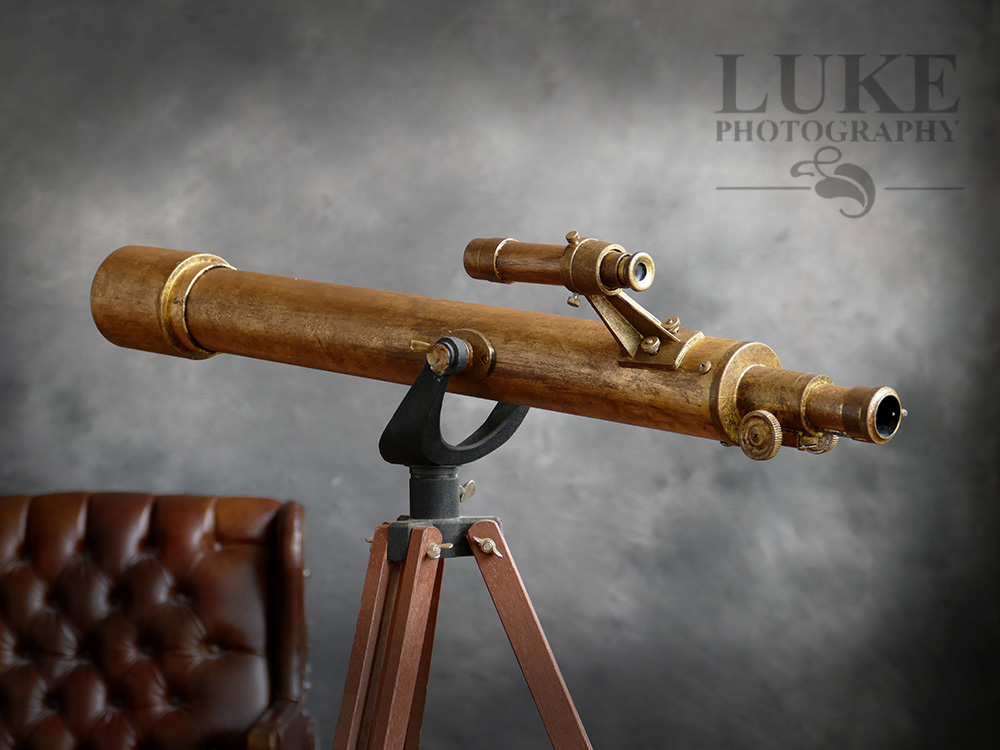The image features a close-up of an antique telescope, exuding a steampunk-inspired aesthetic with its rustic brownish-gold metal body. The telescope is mounted on a black cylindrical holder, which is attached to a robust, triangular base formed by three or four diagonally positioned wooden legs. The intricate setup includes black knobs for adjustments and a secondary, smaller scope mounted on top for enhanced focus. 

Dominating the background is a grey mist-like ambiance, resembling digital fog, which adds a stark, contrasting backdrop to the aged appearance of the telescope. In the top right corner, the text "Luke Photography" is displayed in bold letters with a stylized leaf beneath, enhancing the artistic feel of the image. A dark brown leather chair with buttoned indentations peeks out from the bottom left corner, adding an element of vintage charm to the composition. Overall, the image captures a harmonious blend of nostalgic and modern elements.